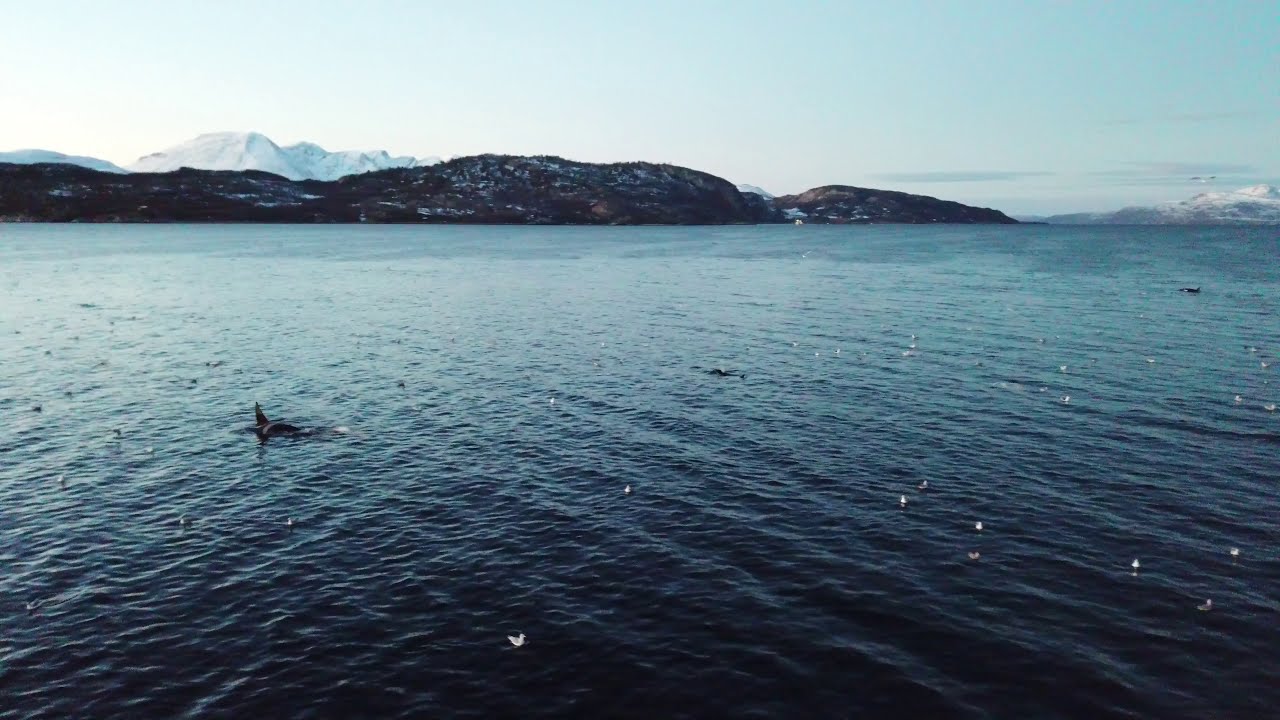The image captures a serene ocean scene dominated by rippling, blue waters that cover about 70% of the picture. Small waves create gentle ripples across the surface. Scattered throughout the water are numerous seabirds, mostly white in color, including seagulls both floating and in flight. On the left side of the water, a dorsal fin rises prominently, suggesting the presence of a large marine mammal, likely a killer whale. A similar dorsal fin appears in the distant right, further hinting at whale activity. In the center, a blowhole is visible, possibly belonging to another whale. The top third of the image showcases a picturesque background with a town nestled in rolling hills, leading up to towering, snow-capped mountain peaks on both the left and right sides. The sky above is clear and blue, with a warm light suggesting late evening sun from the left. The setting, with its mountainous backdrop and abundant marine life, evokes the coastal regions of Washington State, such as the Puget Sound, known for its whale sightings.